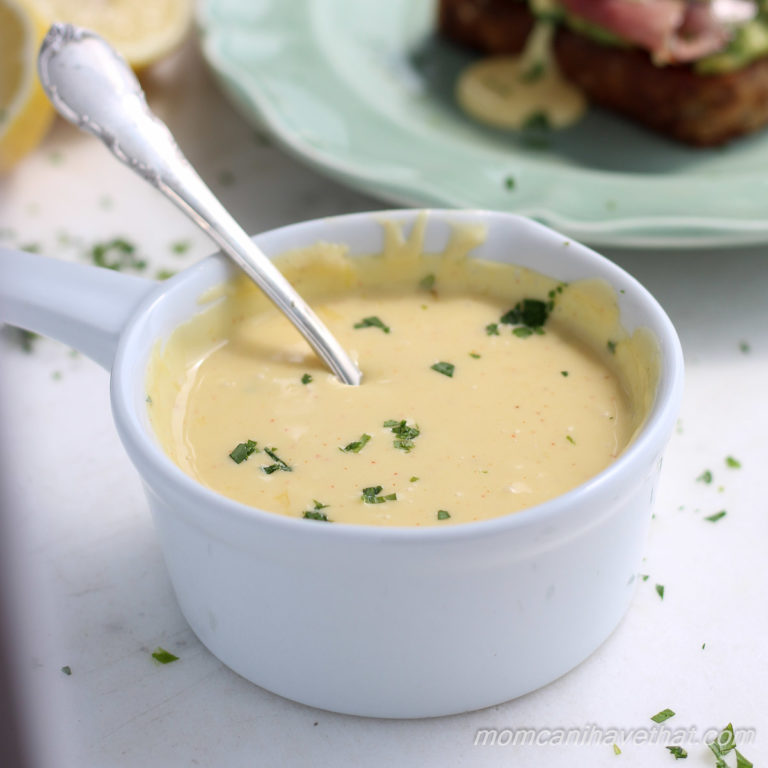The image features a close-up of a white bowl with a handle extending to the left. The bowl contains a creamy, yellow sauce or soup, possibly cheddar-based, that is garnished with green flecks of parsley or chives. A silver spoon is angled out of the bowl to the left. The bowl rests on a pristine white table or tablecloth. In the background, slightly blurred, is a green ceramic plate with a portion of food that appears to be drizzled with the same yellow sauce, suggesting it might be a hollandaise or bearnaise sauce. The food on the plate might include a small piece of steak or potato, with a potential garnish on top. Additionally, the top left of the image features out-of-focus lemon wedges. Finally, there is overlay text on the bottom right corner that reads "MomCanIHaveThat.com".